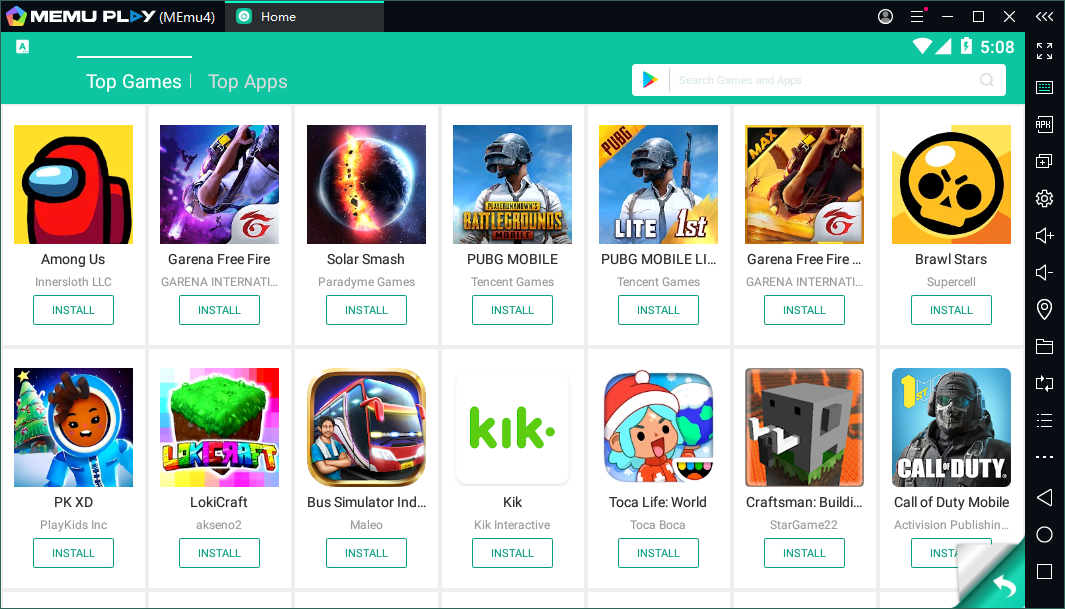Screenshot of a computer screen displaying the MEmu Play interface for downloading games. At the top, a black bar spans the screen with another black bar extending down the right side, each featuring various menu options. Below the top black bar is a thicker turquoise bar with the title "MEmu Play (MEmu-4)" and a home button next to it. Within this turquoise bar, there are tabs labeled "Top Games" and "Top Apps."

The main section of the screen is divided into rows and columns showcasing different game options. There are two rows, each containing seven rectangular tiles. Each tile represents a different game, featuring a promotional image or logo, the game's name, the developer's name, and an "Install" button below each game description. On the top left, the first game displayed is "Among Us," while "Call of Duty Mobile" is positioned at the bottom right of the displayed games. 

To navigate through more game options, there is a small turquoise arrow button at the bottom right corner of the screen, indicating the availability of additional pages. The black bar on the right side of the screen contains multiple buttons for adjusting various settings.